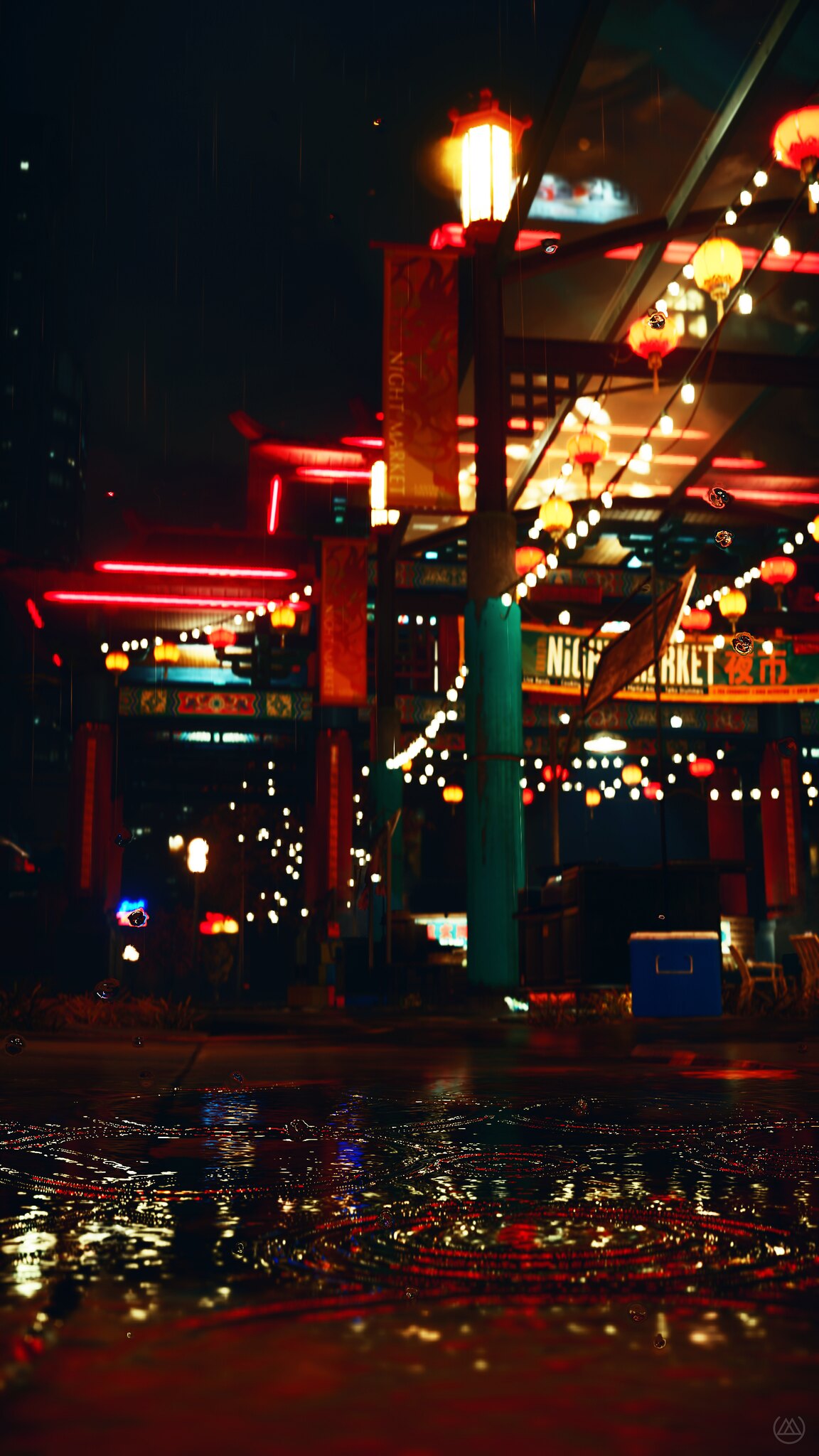The nighttime cityscape reveals a vibrant scene, likely in an Asian country, characterized by a wet, reflective street surface that hints at recent rainfall or possible flooding. The sky above is pitch black, contrasting dramatically with the riot of colors below. Dominating the scene is a teal lamppost stretching nearly vertically through the center, accompanied by a red pole in the distance. Strings of glowing white lights, interspersed with orange and yellow hues, festoon the air between these poles, creating a festive canopy. Alongside these, multiple lanterns cast a warm, inviting glow in shades of yellow and red.

In the mid-ground, a rooftop is adorned with horizontal pinkish-red neon lights, while orange banners flutter gently, attached to various poles and lampposts. The upper part of a market sign is partially visible, with the letters "K-E-T" discernible amidst a backdrop of Asian script, suggesting the locale’s cultural context. Near the bottom of the scene, a blue cooler sits on what appears to be an outdoor porch, further grounding the image in a market or restaurant setting, bustling yet serene in the night’s embrace.